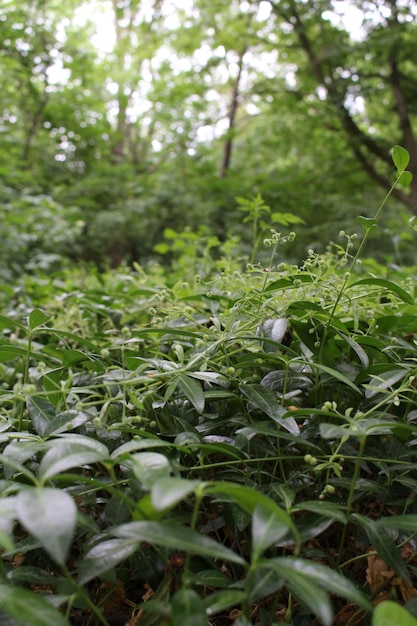This photograph captures a lush forest floor teeming with vegetation. Dominated by green hues, the ground is carpeted with thick, spiky plants, some of which bear white buds, while others seem to have small green sprouts. These plants, perhaps crabgrass or weeds, are very detailed and in focus, giving a vivid texture to the foreground. Surrounding this greenery are numerous bushes and shrubs, creating a heavily covered scene that leaves no bare ground visible. In the background, a dense array of tall trees with slender, brown trunks and thick clusters of green leaves soar upwards. Sunlight filters through the foliage, creating dappled patterns on the forest floor and suggesting a sunny, summer day. Towards the front of the image, a subtle hint of brown from dried fallen leaves adds a touch of contrast to the otherwise predominantly green scene. The sky appears white, likely due to bright sunlight, which further enhances the lively and vibrant atmosphere of this natural setting.